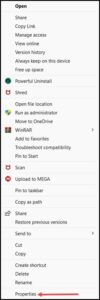This image, enclosed by a solid black border, is a vertically oriented rectangle. The entire picture is out of focus, rendering the predominantly black text within it faded and blurred, making it challenging to decipher. Words such as "copy line," "marriage," "powerful," and "uninstall" are somewhat detectable, although much of the text remains indistinct.

The composition includes several symbols positioned either on the far right or far left of the page. One notable symbol is a dark-colored circle, followed by another circle containing a red symbol. A third circle features multiple colors, including green, blue, and yellow. Additional discernible text reads "WinRAR," "add to favorites," "pin to start," "copy," "share," "cut," and "copy" again.

At the very bottom left corner of the image, the word "properties" is visible. A prominent red arrow points to this word from near the bottom right corner, directing attention across the page. Despite these elements, the overall blurriness makes the finer details and other text difficult to make out clearly.